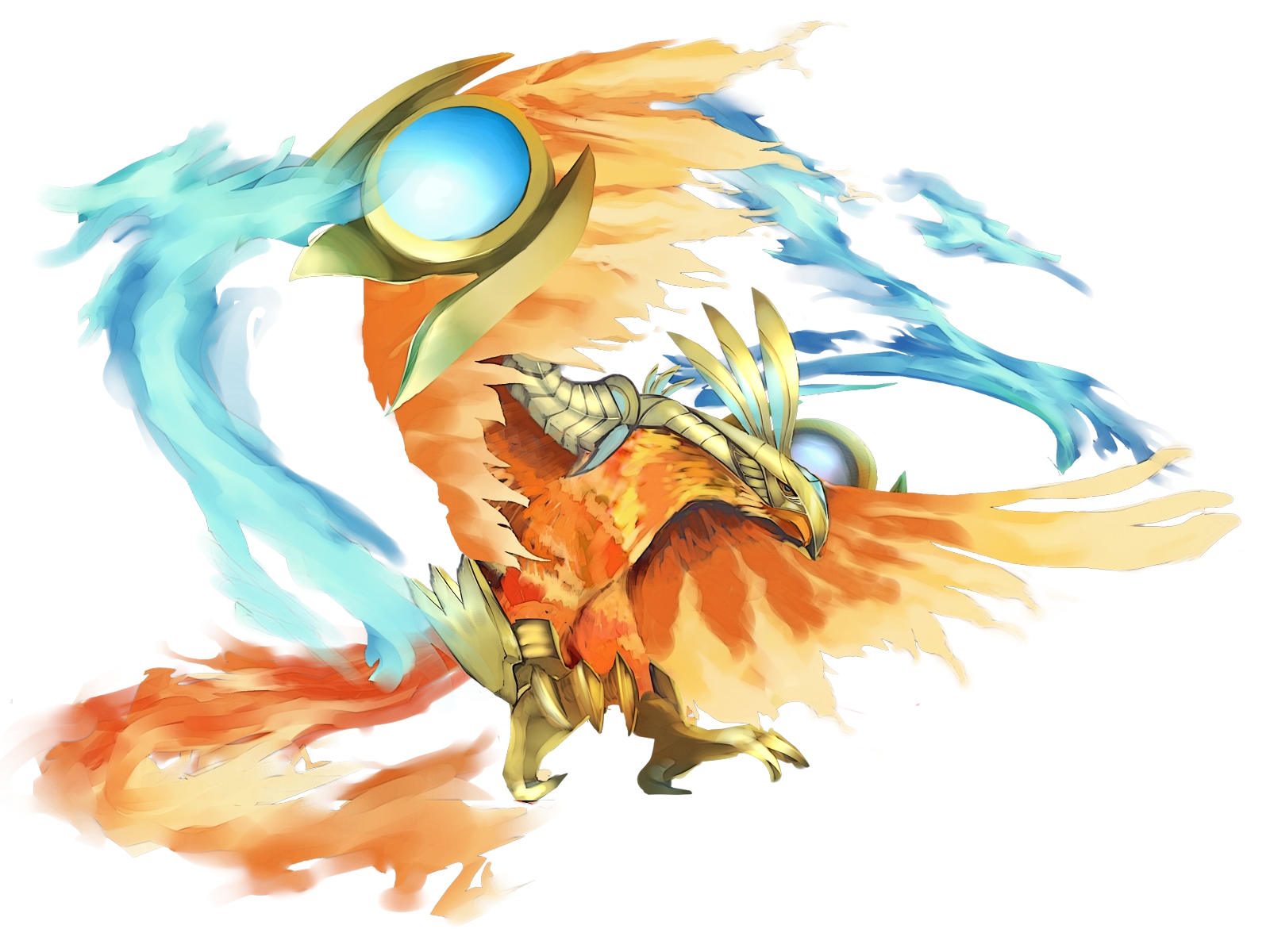The image depicts a detailed, hand-drawn phoenix characterized by its vibrant colors and intricate design. The phoenix has a body and feathers predominantly in shades of orange, which transition to a lighter hue towards the tips of its wings. It bears an almost majestic appearance with a shield-like adornment on its head and right arm. Its talons are vividly poised as if it's about to land, creating a dynamic pose. Surrounding the phoenix, a series of blue swirls and designs add a contrasting backdrop, while an abstract, multi-colored watercolor pattern enriches the background, predominantly featuring orange hues. The overall scene is vivid and lively, capturing the essence of a mythical creature in motion.